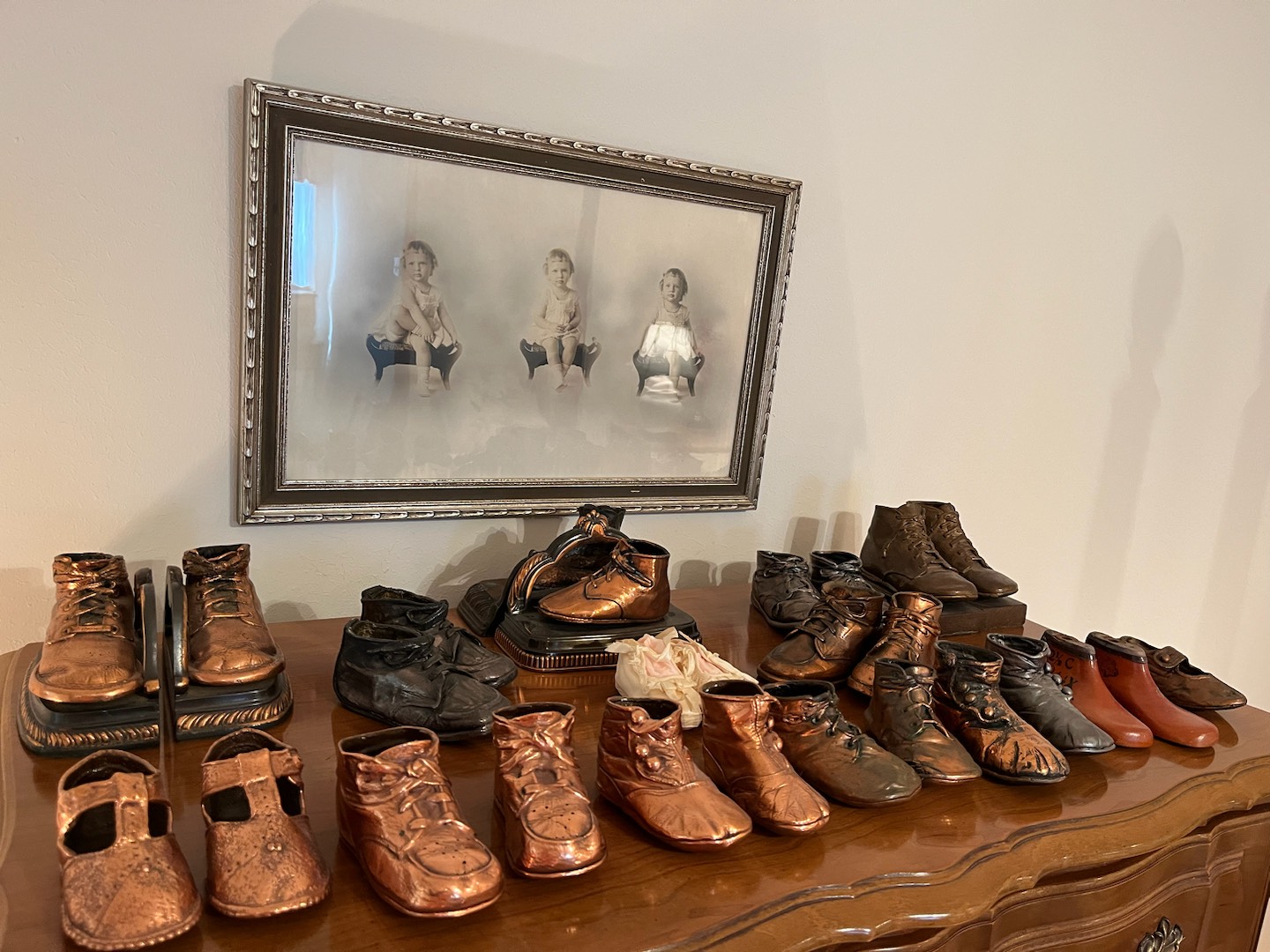The horizontal rectangular image depicts a collection of bronze and copper-colored baby shoes, arranged meticulously on an ornate wooden dresser. These pairs of shoes, various in styles and placed both on the front of the dresser and on books or pedestals towards the back, create a visually captivating scene. Above the dresser, hanging on the white wall, is a silver ornate frame housing a trio of black-and-white baby photographs, likely of the same child. The matting of the frame is white, complementing the overall aesthetic. Reflections on the glass of the frame hint at a well-lit room or light sources nearby, enhancing the detailed display of shoes that transition in color from vibrant bronze on the left to more leathery hues of brown towards the right. This careful arrangement underscores a nostalgic homage within a sophisticated setting.